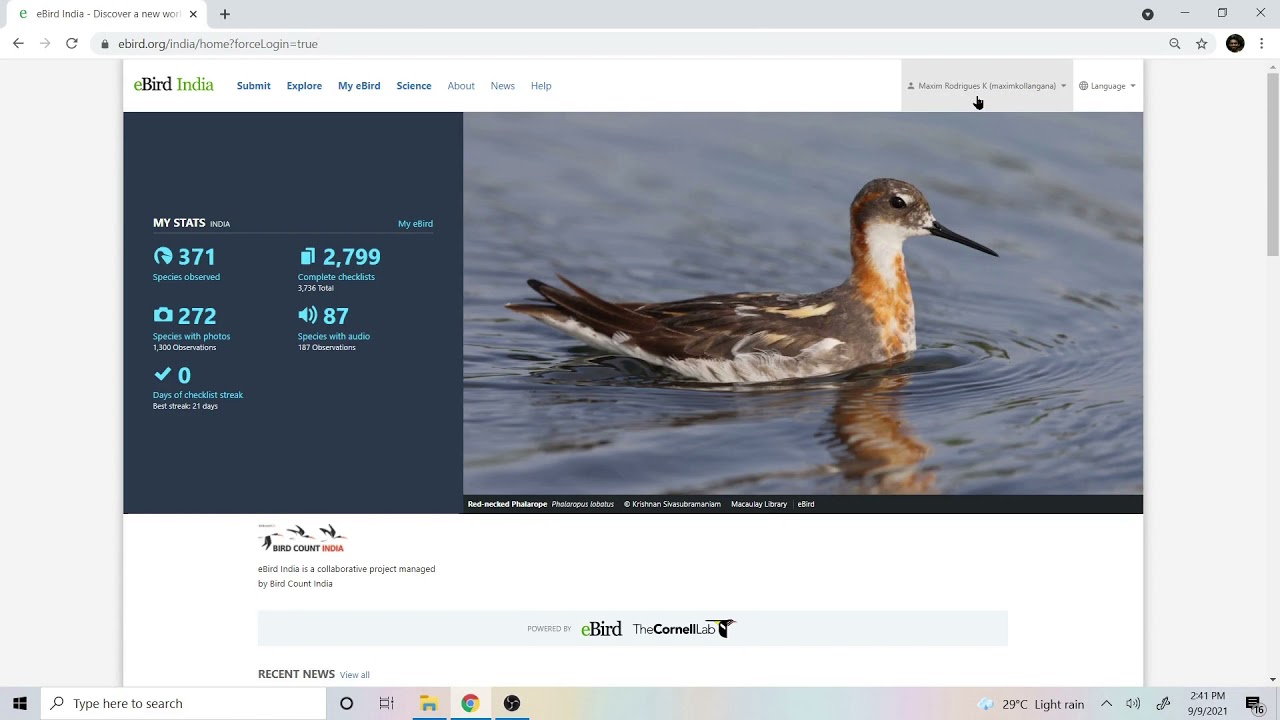This detailed screenshot captures the eBird India website as displayed on a computer screen. In the top left corner, a single tab is open labeled "eBird India," accompanied by a small 'X' to close the tab. Adjacent to it on the right is a plus sign for opening new tabs. On the far right, the typical window control buttons - minimize, expand, and close - are visible.

Dominating the central part of the page is the "eBird India" title, flanked by navigational links including "Submit," "Explore," "My eBird," "Science," "About," "News," and "Help." On the left-hand side is a "My Stats" section. Featured prominently within this section is a clickable "My Edited" button, followed by several statistics: 
- 371 species observed
- 2799 complete checklists
- 172 species with photos
- 87 species with audio
- 0 days of checklist streak

Below the stats, the image showcases a photograph of a bird with a long, narrow beak, floating on water. The bird is adorned with a mix of gray and white feathers on its head, back, and under its neck, while its chest boasts rust-colored feathers. Underneath this visual, the text reads "BirdCount India." It further indicates that eBird India is managed collaboratively by BirdCount India and is powered by eBird and the Cornell Lab.